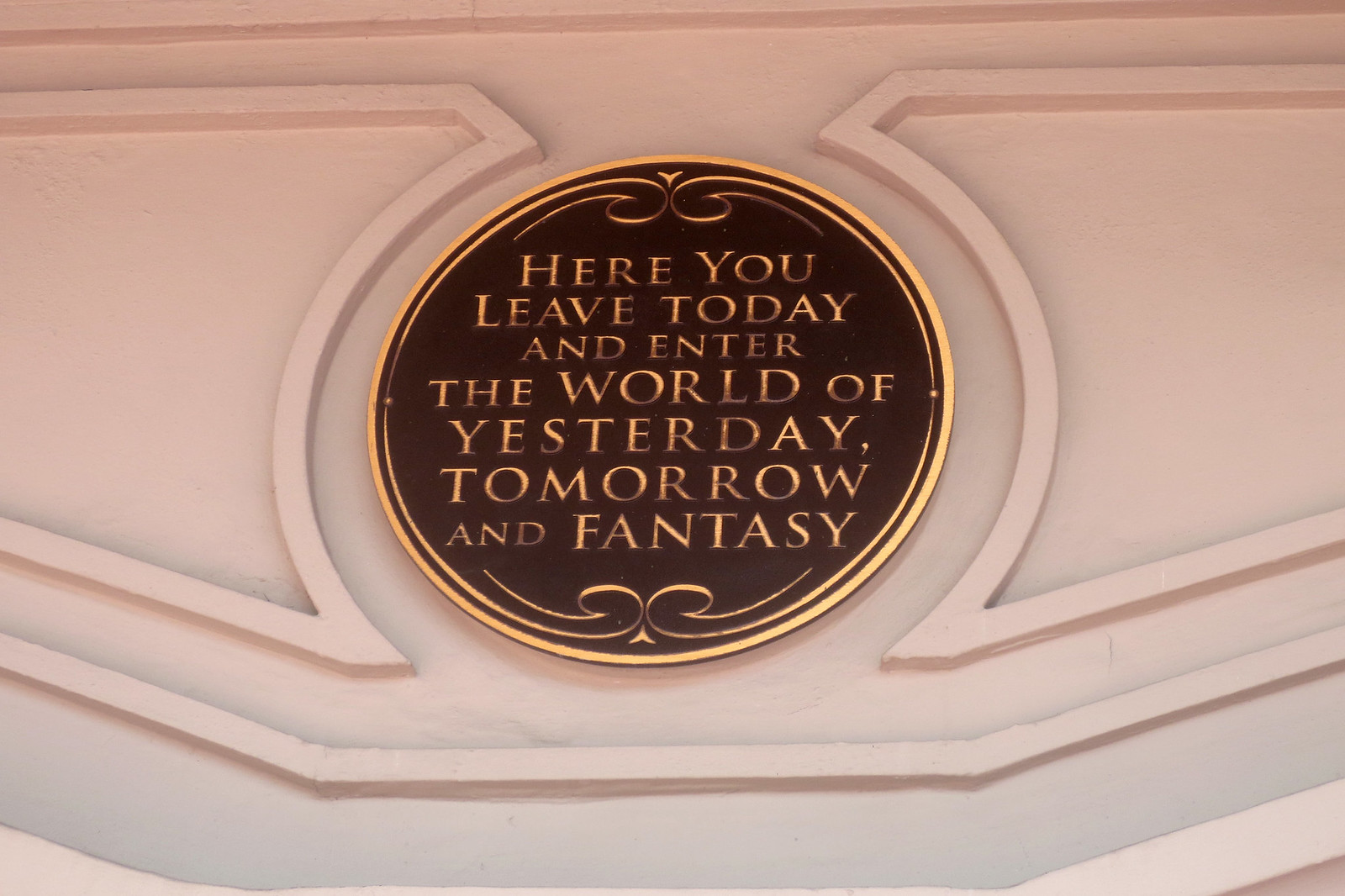The image depicts a plaque mounted above what appears to be a doorway, possibly at the entrance of a building. The plaque is oval in shape with a dark brown or black antiqued center and a gold outer rim that adds a decorative touch. The text on the plaque, written in elegant gold letters, reads: "Here you leave today and enter the world of yesterday, tomorrow and fantasy." The plaque is framed by raised, symmetrical design elements on the wall that create a circular pattern around it. The photograph itself has a pinkish tint, adding a vintage or whimsical feel to the scene. The overall setting suggests it could be part of a grand entrance, possibly within a school, college, or even an exterior façade welcoming visitors to a special place.